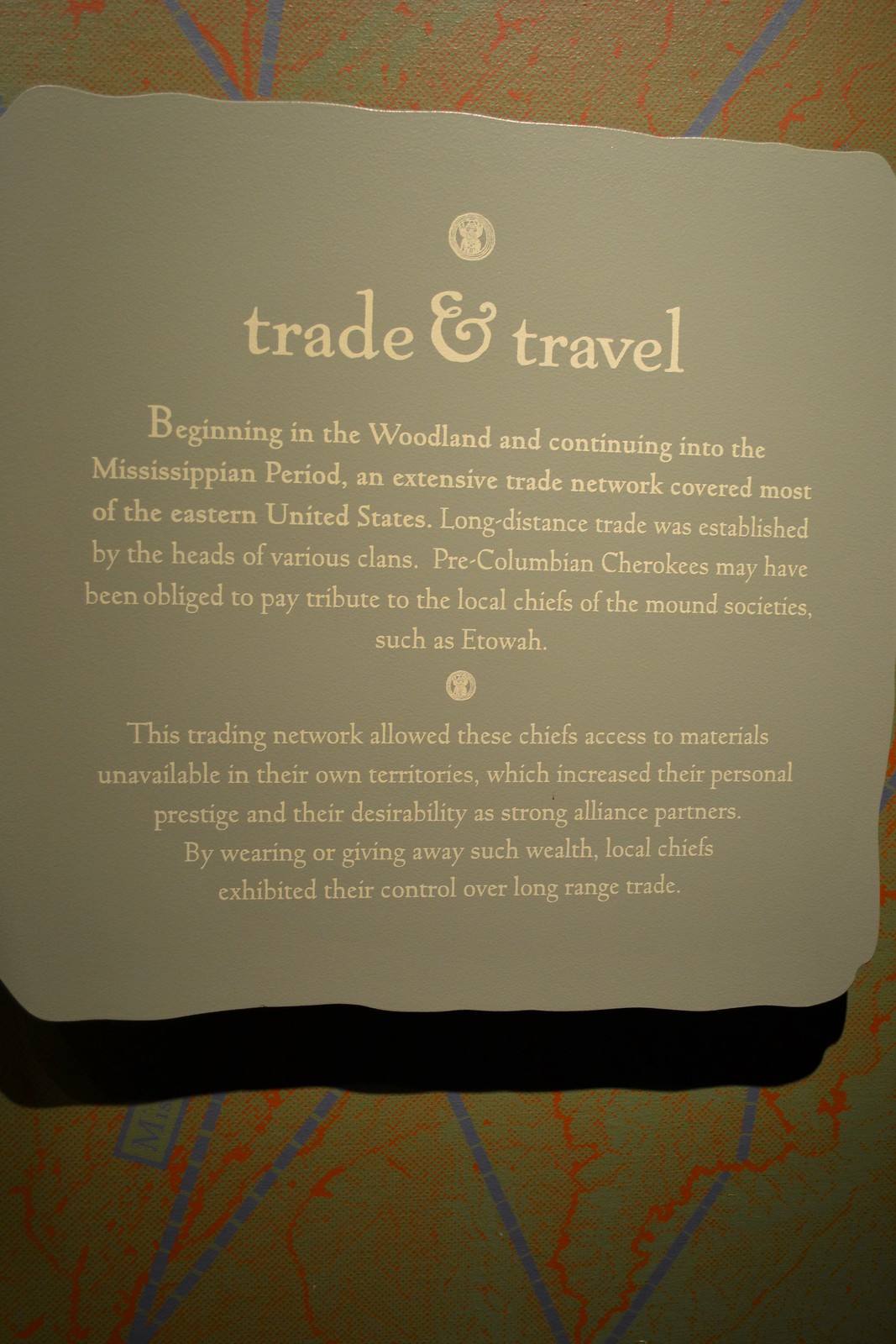The image features a museum display sign mounted on an olive green wall adorned with a striking pattern of blue and orange stripes. The sign has a dark tan background interspersed with diagonal and vertical blue, orange, and green lines, contributing to a vibrant, intricate design. At the top of the sign, an emblem or logo is present, followed by the bold heading "Trade and Travel" likely written in tan or peach letters. The text on the sign explains that, beginning in the Woodland period and continuing into the Mississippian period, an extensive trade network covered much of the eastern United States. This network was formed by the heads of various clans who established long-distance trade, gaining access to materials not available in their own territories and thereby increasing their prestige and desirability as strong alliance partners. This historical insight suggests the sign is meant to contextualize a nearby exhibit, possibly related to Pre-Columbian Cherokee societies and their tribute-based trading systems.